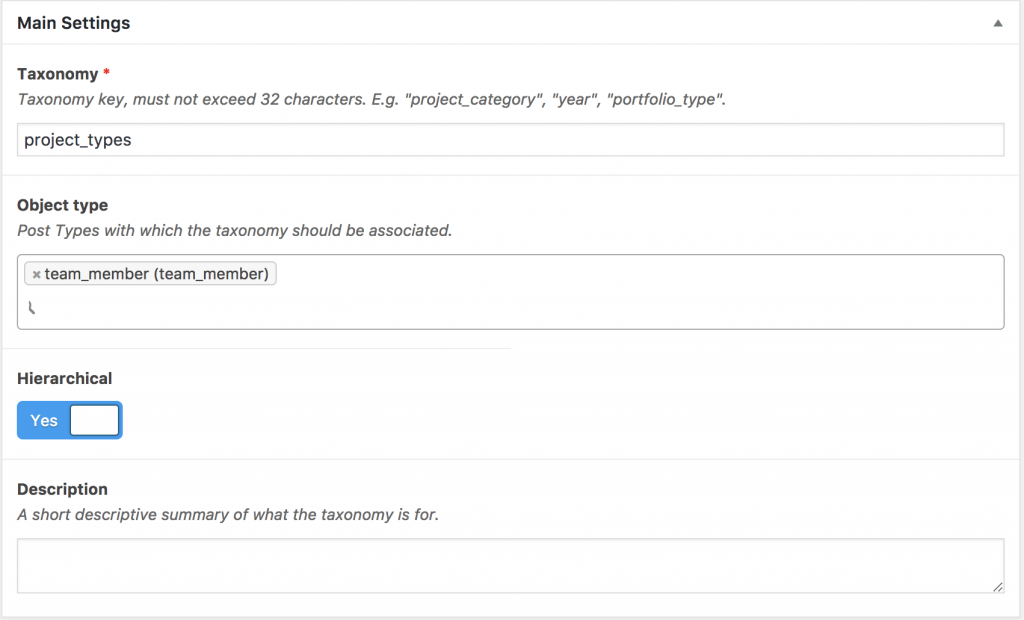The image shows a user interface screen with a white background and black text, designed for configuring main settings. At the top left, it prominently displays "Main Settings." Directly below this heading is a section titled "Taxonomy," which includes a guideline stating, "Taxonomy key must not exceed 32 characters, e.g. project_category, portfolio_type." Underneath this guideline is an input field labeled "Taxonomy," where "project_type" is currently entered. 

To the right of the input field, there is a red asterisk indicating that this field is mandatory. The next section is labeled "Object Type," accompanied by a description: "Post types with which the taxonomy should be associated." One object type is selected in this area, displayed as "team_member (team_member)." 

Following the object type selection is a blue toggle switch, which is white in the center and labeled "Hierarchical." The switch is set to "Yes." Beneath this toggle switch is a section for "Description," which prompts the user to provide a short descriptive summary of the taxonomy's purpose. This field is currently empty. The entire setup features a clean, white background with black text, ensuring clarity and readability.